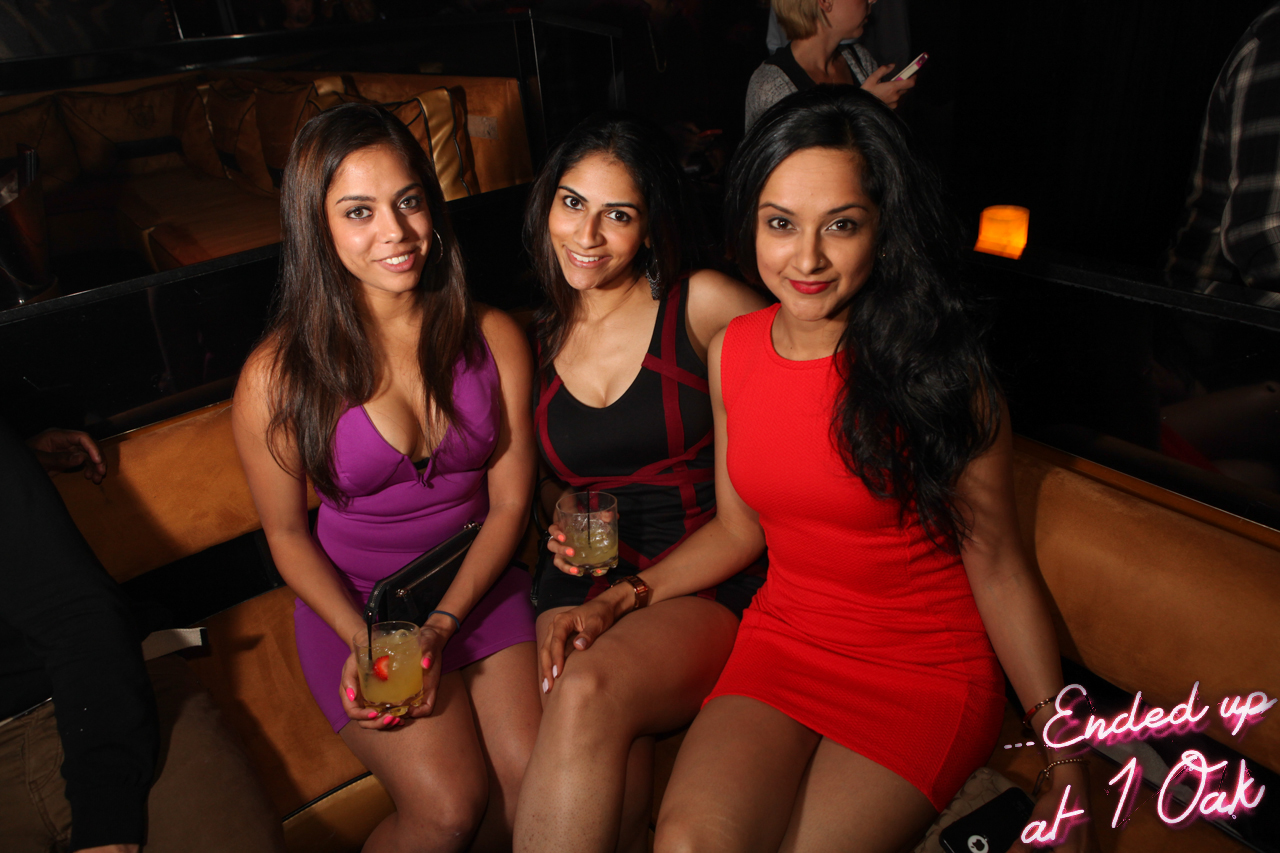In this detailed photograph, three young women, dressed in tight, short dresses typically worn in a club, are seated closely together on an L-shaped, suede leather-type sofa. The woman on the left is wearing a low-cut purple dress and holding a yellow drink in her hands, with a black clutch resting on her lap. She has long, dark hair and dark eyes. In the middle, another woman also with long dark hair and dark eyes, is in a black dress with red lines, also holding a similar drink. The woman on the right is wearing a short, red dress, featuring long dark hair, dark eyes accentuated with red lipstick, and has her hand placed on the middle woman's leg. All three are smiling as if posing for the picture. The background is dimly lit but reveals other people and a secondary lounge area with a similar sofa. A woman can barely be seen standing behind them, with a phone in her hand. Additionally, a light or electric heater emitting an orange glow is partially visible. At the bottom right corner of the photograph, shiny pink letters spell out "Ended up at One Oak."